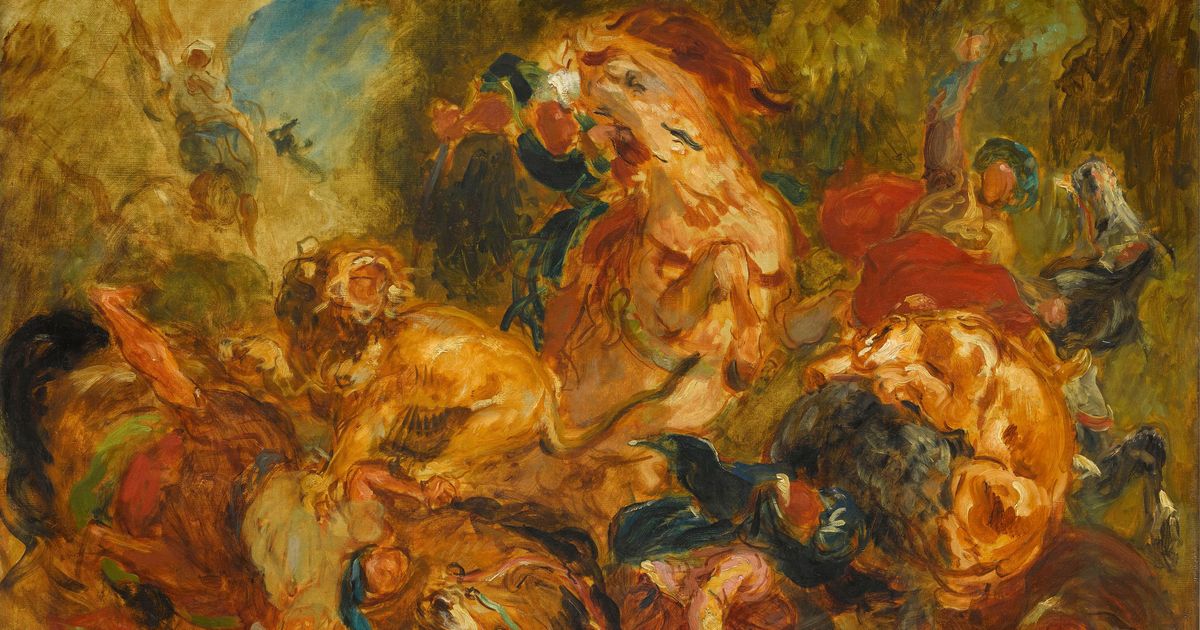This intricate painting, possibly a famous masterpiece, depicts a chaotic and somewhat abstract battle scene. The medium is likely oil on canvas, evident from the blending and texture of the brush strokes. An array of colors dominates the composition, including browns, beiges, greens, oranges, rusts, dark blues, and vibrant yellows, melding together to form a cohesive yet ambiguous image.

At the heart of the painting, a tumultuous clash unfolds amidst a wooded landscape marked by tree trunks and traces of blue sky. Central to the scene is the vague but discernible figure of a rearing horse, surrounded by men riding and falling from other horses. The fragmented forms and shades suggest a myriad of creatures, including lions with distinctive manes, a black bird, and perhaps other beasts engaged in combat. Faces and figures emerge sporadically within the chaos, with one individual possibly wearing a turban.

In the lower parts of the painting, more gruesome details come into view: a partially devoured person and a face on the ground, intermixed with fur, feathers, and unidentifiable objects. The inconsistent, blotchy, and blurry visual presentation enhances the sense of hyperactivity and confusion, characteristic of a battleground.

Overall, this artwork employs a dynamic color palette and abstract forms to depict a fiercely violent scene with both human and animal participants, leaving much to the viewer’s interpretation.